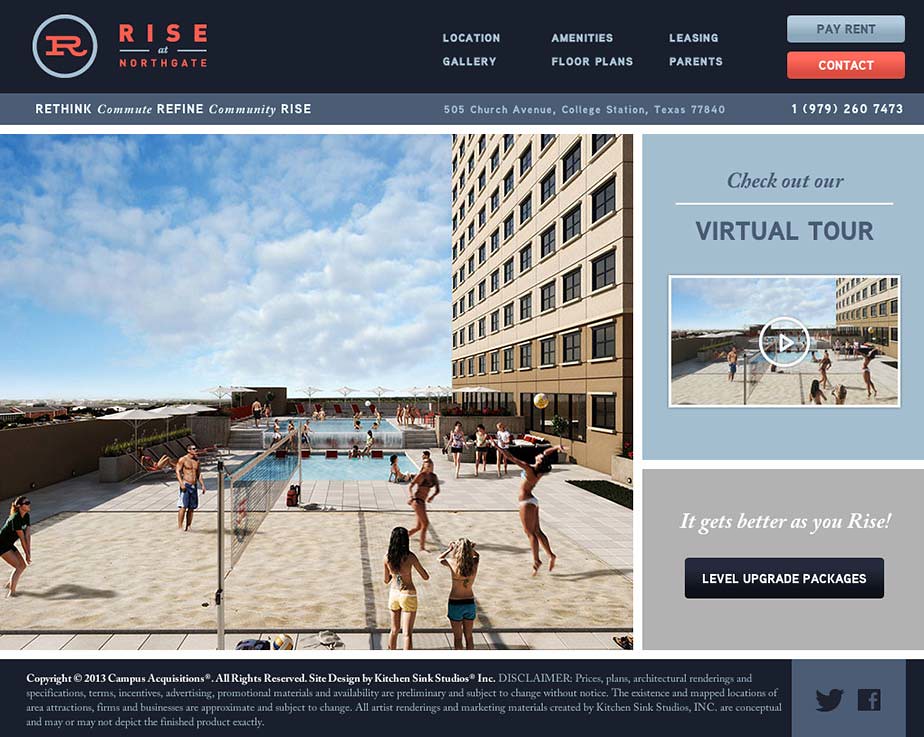This image is a screenshot of a website for an apartment building named "Rise at Northgate." Dominating the top-left corner is a logo featuring a light grey circle with a red "R" and the text "Rise at Northgate" in red. Adjacent to this are clickable options including Location, Gallery, Amenities, Floor Plans, Leasing, Parents, as well as buttons for Pay Rent and Contact situated on the far right. Below the header, a dark grey band displays the text: “Rethink, Commute, Refine, Community, Rise,” along with the address "505 Church Avenue, College Station, Texas, 77840-1979-260-7473." Following this, the main visual content centers around a large photograph to the left, depicting an outdoor area of the apartment complex. Prominently visible is a recreational area with a rooftop pool that features a cascading waterfall into a smaller pool. Adjacent to the pools is a sandy volleyball court where several people are actively playing, including women in bikinis and others in swim trunks, with onlookers nearby. On the right side of the image, there is an option to check out a virtual tour, accompanied by the text "It Gets Better As You Rise" and a button labeled "Level Upgrade Packages." At the bottom, the site provides copyright information and clickable icons for Twitter and Facebook.